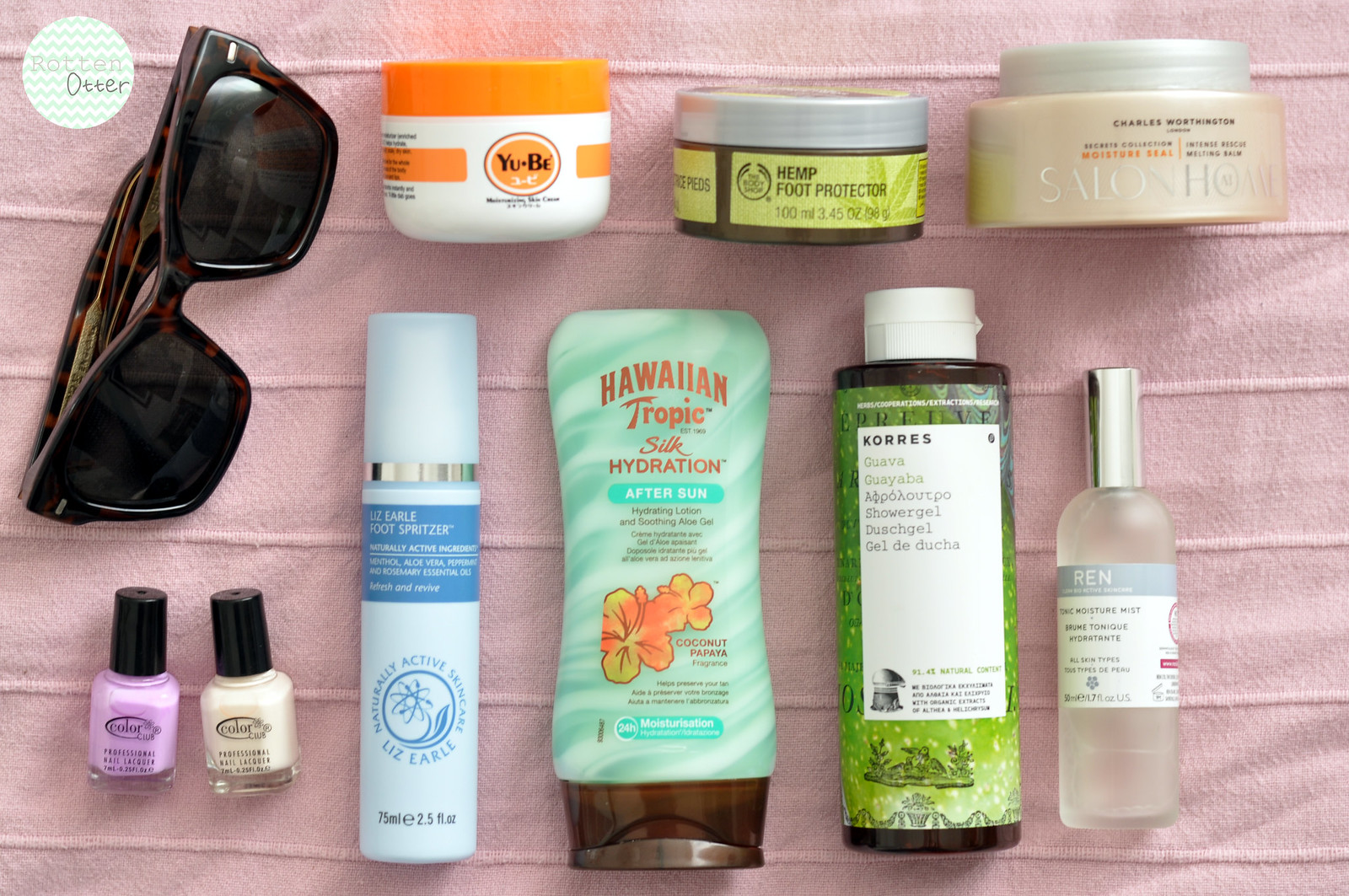In this image, a series of different products are meticulously arranged on a light purple towel, providing a soft, textured background. The towel features six evenly spaced horizontal lines that form subtle rows and contribute to its design. 

In the bottom left corner, two nail polish bottles sit side by side; one is light purple, and the other is white, both sporting black caps. Moving to the right, there is a light blue bottle adorned with a matching blue label. Continuing rightward, a bottle of Hawaiian Tropic Silk Hydration After Sun lotion catches the eye with its light blue and white striped pattern, complemented by yellow and orange flowers at the bottom and a dark brown base.

Next, there is a bottle with a green background, a white label, and a white cap, followed by a clear bottle with a white label and silver cap. Above these items, a wide-based container is positioned, and to its left, a slightly smaller container labeled "Hemp Foot Protection" with a gray cap. Further left, there is a small orange and white container.

In the top left corner of the image, the logo "Rotten Otter" is prominently displayed within a white circle, adding a touch of brand identity to the composition.